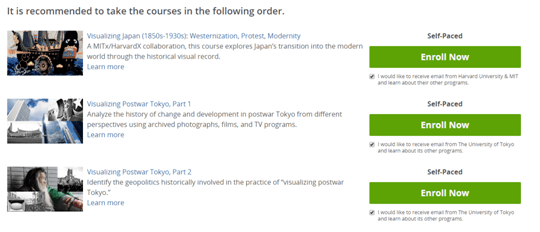"Screenshot of an online education webpage displaying recommended course sequence and enrollment options. At the top, in black font, the text reads: 'It is recommended to take the courses in the following order.' The page lists three courses side by side, each accompanied by a photo. To the left of each description, there's a small, color stock image for the course. 

The first course is 'Visualizing Japan, 1850s: Westernization, Prada, and Modernity.' The description is paired with a green 'Enroll Now' button in white font, overlaid with 'Self-paced' in black. Below the button, an option reads: 'I would like to receive email from Harvard University and MIT and learn more about their programs.'

The second course, 'Visualizing Post-War Tokyo, Part 1,' has a similar setup. The 'Enroll Now' button and the email preference text change to: 'I would like to receive email from the University of Tokyo.'

The third course, 'Visualizing Post-War Tokyo, Part 2,' maintains the same layout and email preference as the second course.

The overall design is clean, though the image is slightly blurry due to zooming in, making some details hard to discern clearly."